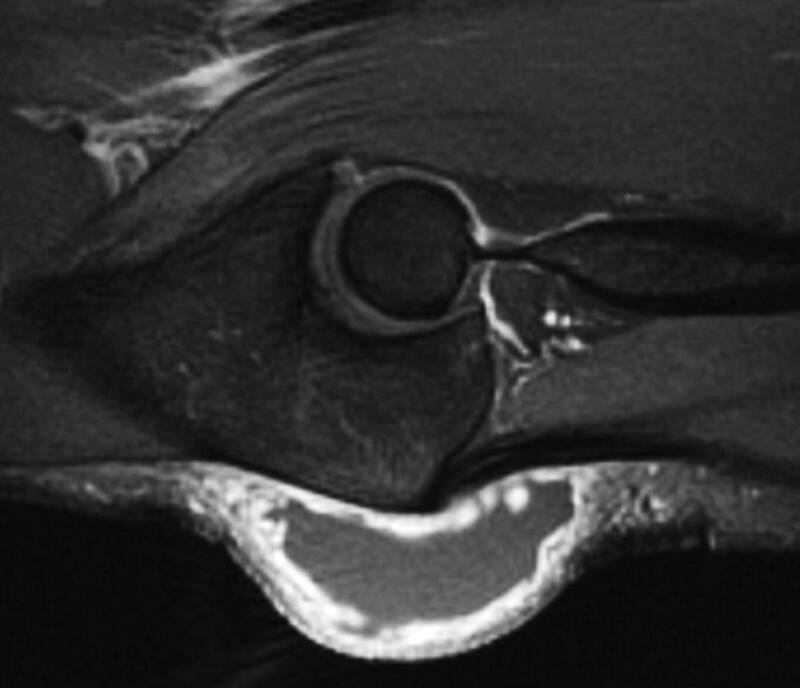This image, likely an ultrasound or x-ray, is captured in a grainy black-and-white format, resembling a square landscape orientation. At the top left corner, there's a distinct illumination, almost reminiscent of a wave crashing, characterized by a bright white light. The center of the image features a circular shape with a white border, surrounded by a different textured tissue, and showing some dark streaks extending to the right. Below this circle, the bottom of the image exhibits a bean-shaped or smiley face formation, also brightly lit along its perimeter. This particular area is described as having a resemblance to an open human mouth with a visible canine and a gum line, but it's clear that the interpretation of anatomical features is subjective and unclear. The darker areas and various swirling textures add to the complex, abstract nature of the image.